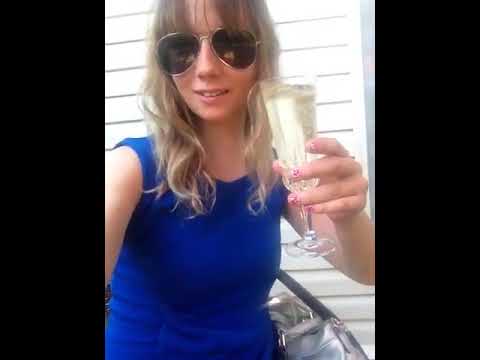The image, framed by thick black borders on the left and right, features a woman in a blue sleeveless dress with shoulder-length blonde hair, styled with bangs. Her head is slightly cut off at the top by the frame. She is facing forward but slightly turned to her right, with a faint smile that reveals her top row of teeth. Her eyes are partially visible through large aviator sunglasses with silver frames and brown-tinted lenses. In her left hand, which is adorned with pink nail polish, she holds out a champagne glass containing a clear or light-colored liquid. Her right arm is cut off at the upper arm by the edge of the image, possibly because she is taking a selfie. A silver handbag is seen by her waist. The background shows horizontal white blinds, suggesting the exterior wall of a building illuminated by bright light. The presence of an edge of a chair can be seen in the bottom right part of the image.